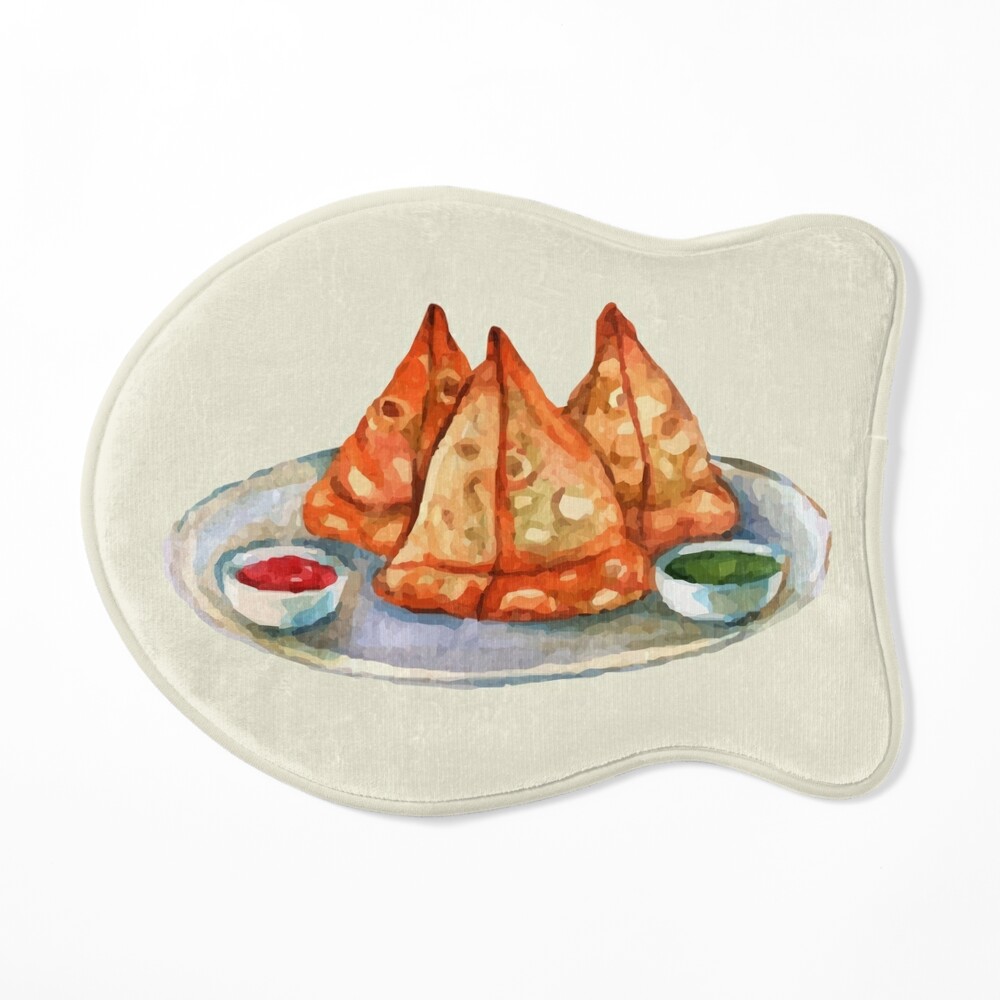In the image, there is a detailed sketch of a dish placed on a plain white background. The sketch is depicted on an item resembling a placemat or cutting board, which is shaped like a cartoonish goldfish swimming to the left, with a rounded circular side on the left and two protrusions on the right. On the sketch, there is a plate prominently displaying three triangular-shaped food items that could be Mexican food like empanadas or Indian samosas, characterized by a light brown and orange, mottled appearance. These items are arranged almost like pizza slices but sitting flat where the crust would be, pointing upwards. Accompanying these are two small bowls of sauces: the one on the left is red and slightly elevated, while the one on the right is green and lays flat within the dish. The green sauce could likely be chutney. The arrangement of these elements on the sketch creates an image that is colorful and rich in detail.